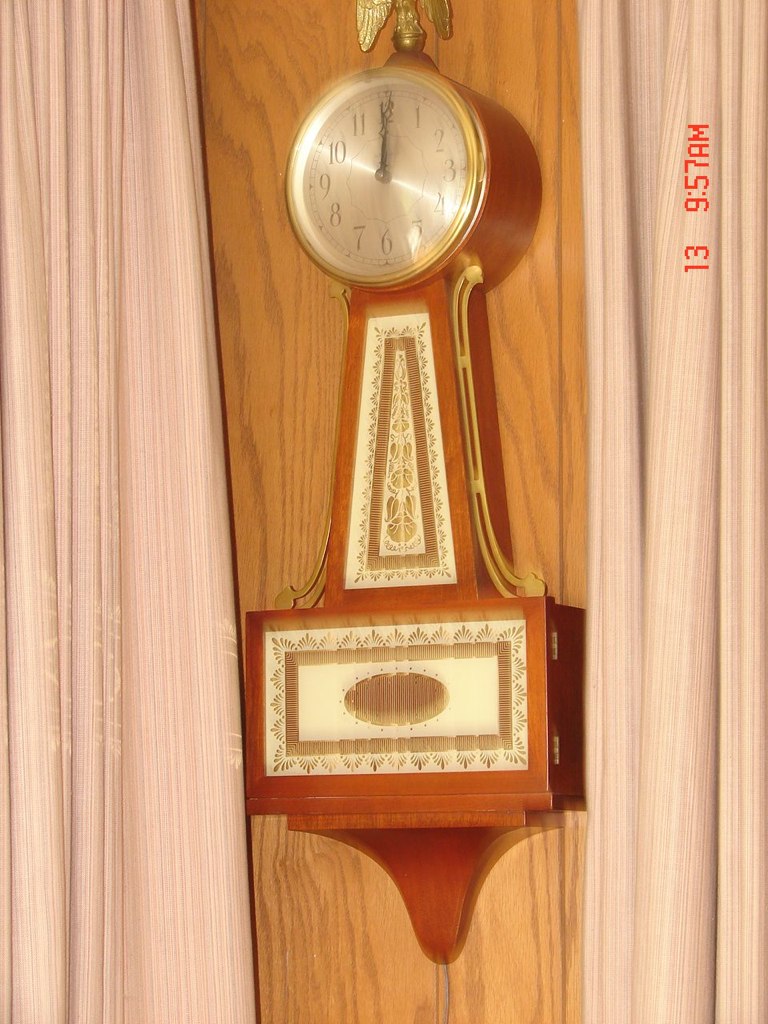The image features a decorative wall clock mounted on wood paneling that is 50% taller than it is wide, divided into three vertical sections. The left and right sections are light-colored wood with defined striations and irregular dips. The center section is a medium brown, slightly darker than the other two sections. 

The clock itself has an analog face, which is silver with a gold circle around it, displaying the time exactly at noon. The clock's design resembles a hammer with a light tan handle and a horizontal rectangular base, all outlined in dark-colored wood. A gold or brass bird figure decorates the top of the clock, with its wings visible, adding a unique touch.

Surrounding the clock, the wood paneling forms a backdrop, complemented by long, white or linen-colored curtains on either side. There are red letters in the top right corner of the image that read "13 9:57 AM," providing a timestamp. Additionally, brass decorative swirls adorn either side of the clock, and the clock's face features simple black numbers.